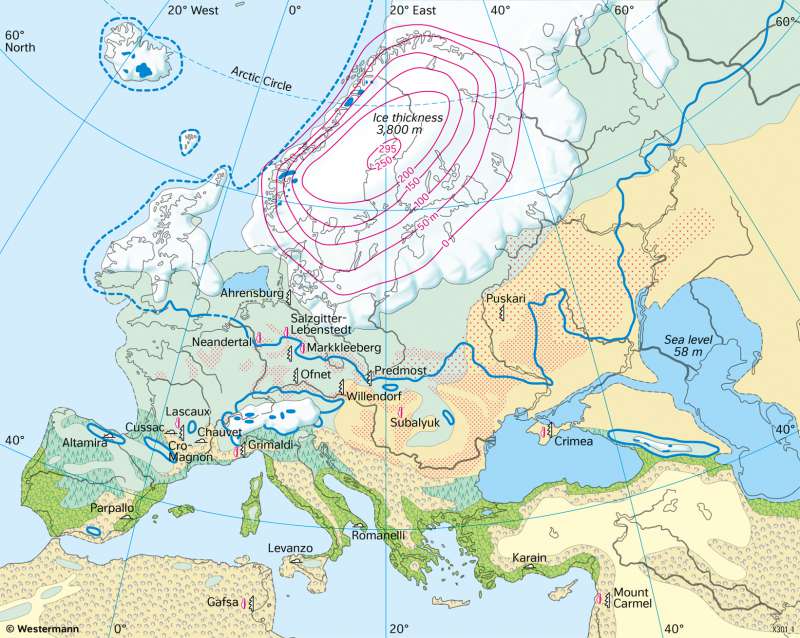The image features a detailed, pastel-colored map encompassing most of Western Europe and the tip of Africa. The map highlights both geographical features and specific measurements, including lines of longitude and latitude in light blue, with prominent markers such as 20 degrees west, 60 degrees north, and 20 degrees east. At the top of the map, a dotted blue line indicates the Arctic Circle, with the land here depicted in white and overlaid by progressively larger ovals and circles in purple, labeled with numbers like 295, 250, 200, 150, down to zero. The map includes bodies of water separating continents, with the bottom left showing Africa and the right depicting regions like Crimea with a marked sea level of 58 meters.

The colors used for the landmasses range from white, pinks, light purples, and light greens to shades of brown and orange, along with gray. Some specific labeled areas such as Ehrensberg, Salzgitter, Lebenstadt, Mark Kleberg, Offnet, Predemost, and Willendorf are included, though they are not recognizable as major cities. Additionally, ice thickness is noted as 3,800 meters.

Overall, this map provides a combination of physical geography with detailed data points, blending aesthetic pastels and functional cartographic details.